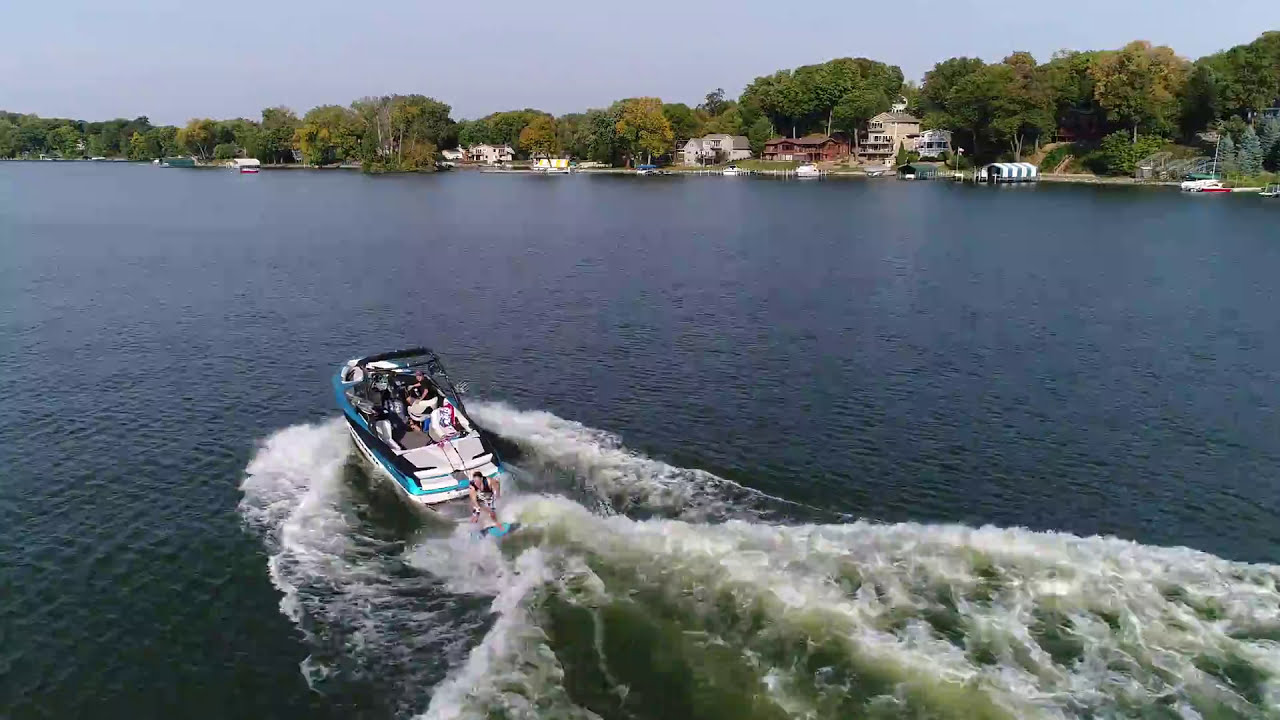This detailed aerial color photograph captures a picturesque lake scene in landscape orientation. The dark blue water of the lake is disturbed by a green and white motorboat moving briskly from the bottom towards the top left of the image. The boat, slightly left of center, creates a wake of large, white frothy waves trailing behind it. A person on a surfboard is being towed by the boat, holding onto a rope and skimming across the water's surface. Another individual appears on the back of the boat, seemingly about to jump into the water. The serene backdrop features a neighborhood lining the lake, with numerous homes, docked boats, and a mix of green and yellowing trees, suggesting late summer or early fall. The pale blue sky above completes the tranquil yet lively composition, emphasizing the realism of this drone-captured moment.